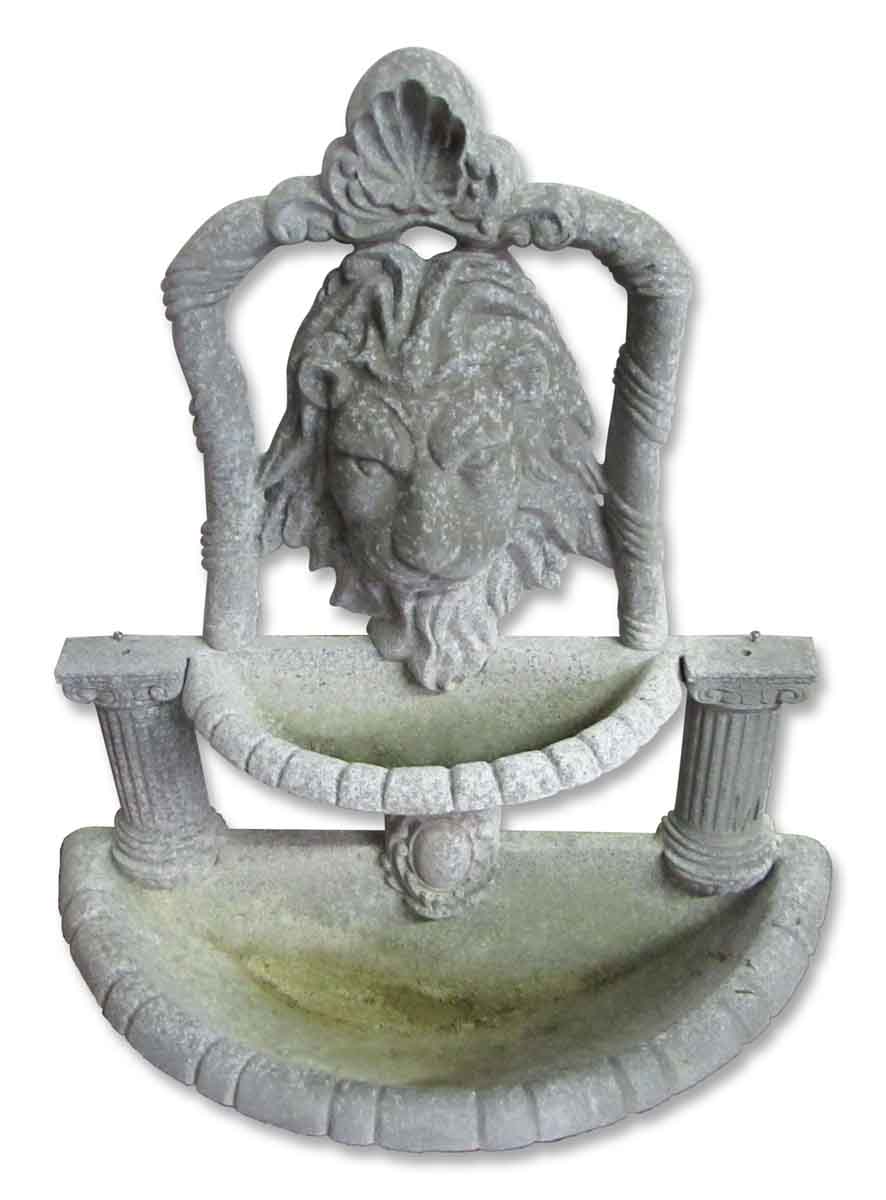The image depicts an ornate water fountain seemingly constructed from gray stone or concrete, featuring a prominent lion's head with a long mane and intense, almost bored expression at the top. The lion's head is set within a decorative frame, possibly flanked by a seashell indentation above it and two columns on either side. The fountain includes two semi-circular basins—one larger at the bottom and a smaller one above it—both adorned with green moss or mildew, indicating they may have once held water. The entire structure is weathered, with greenish hues suggestive of mold growth likely from past water usage. The background is stark white, making the details of the fountain stand out distinctly.